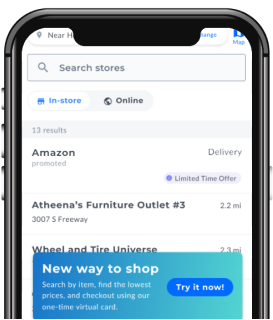In the image, the upper half of a smartphone is displayed on a predominantly white webpage. The phone screen shows a map application that is not clearly identifiable as Google Maps or Apple Maps, possibly suggesting it is a Microsoft app. A prominent search bar at the top of the screen reads "Search stores," but no text has been entered yet. Below the search bar, there are two toggle options labeled "in-store" and "online," with the current setting on "in-store."

In the main content area, three listings are visible. The first is a promoted listing for "Amazon." Following that, there is "Athena's Furniture Outlet," located at 3007 South Freeway, which is 2.2 miles away. The third listing is "Wheel and Tire Universe," situated 2.3 miles from the current location. 

At the bottom of the phone screen, a small advertisement states, "New way to shop. Search by items, find the lowest prices, and check out using our one-time virtual card. Let's try it now." The text on the ad is primarily black with blue elements, contrasting against the white background of the phone's interface.